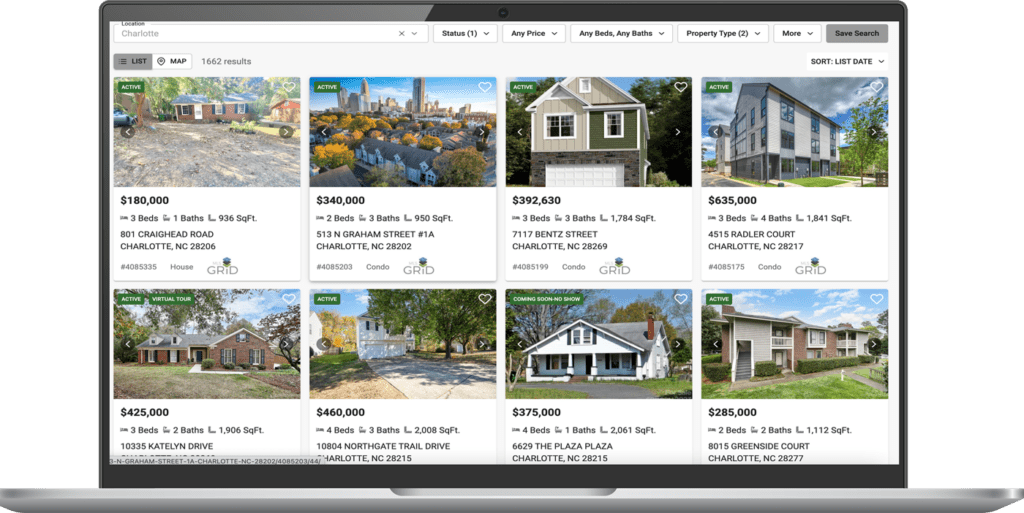The image displays a computer screen with a horizontal rectangular shape, set against a white background. The screen is black both in its display areas and surrounding edges. It is positioned on a sleek silver stand, paired with a wider silver keyboard in front of it. The screen shows two horizontal rows, each containing four vertical rectangular images.

Each image depicts a property listing with details including price, location, and basic features:

1. The first image in the top row shows a small house on a property, priced at $180,000, with three bedrooms and one bathroom, located in North Carolina.
2. The second image features another property in Charlotte, North Carolina, listed at $340,000.
3. The third image showcases a house with tan siding and white molding, priced at $392,630.
4. The fourth image captures a light-colored house, listed at $635,000.

In the bottom row:

1. The first image displays a house with dark siding and shutters on the windows, priced at $425,000.
2. The second image is less clear but lists a property priced at $460,000.
3. The third image shows a small white house, priced at $375,000.
4. The fourth image depicts a tan house, listed at $285,000.

All properties are located in Charlotte, North Carolina. The images are somewhat small, making some details hard to discern.